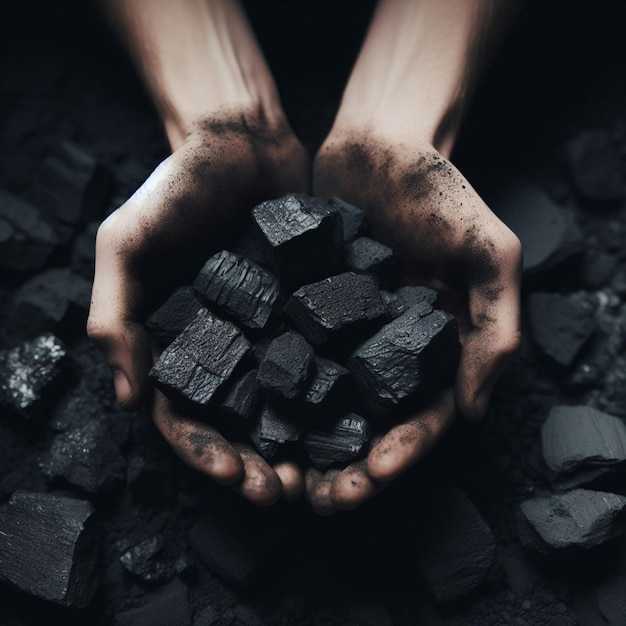This detailed image captures a pair of cupped, Caucasian hands emerging from the top of the frame, holding irregularly shaped chunks of charcoal. The hands, which are textured and dusted with charcoal powder, frame the matte black and sometimes shiny pieces nestled within the palms. The background transitions from a solid black near the wrists to a dispersed scattering of larger charcoal chunks below, enhancing the contrast between the light skin and the dark elements. The focus is on the charcoal, which dominates the image with its varied shapes and subtle glitter, while the blurred arms and dark background emphasize the central theme of the coal-stained hands.